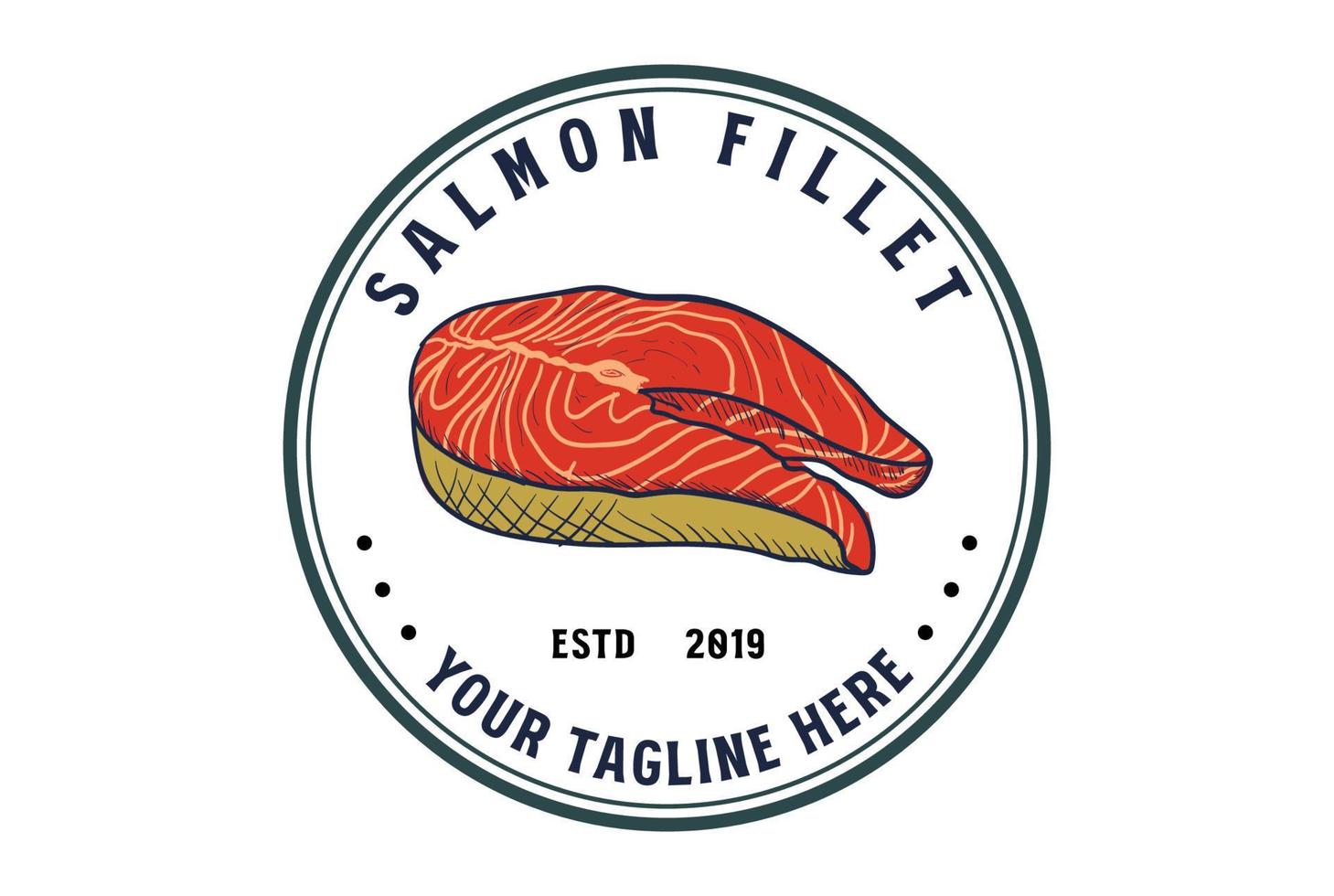The image displays a logo set against a plain white background, dominating the scene. The logo itself is circular with a black border, followed by another inner black line that encloses a white central area. At the top of the circle, in black text, it reads "Salmon Fillet." Below this, centrally placed, is a cartoon-like depiction of a salmon fillet, characterized by its red interior and a yellowish-tan outer skin, shaped somewhat oval or akin to a bird’s beak. Below the salmon image, in black text, are the words "ESTD 2019." Further down, separated by three small, dark dots on either side, is the placeholder text "…your tagline here…," also in black. The simplicity of the background emphasizes the clarity and details of the logo design.